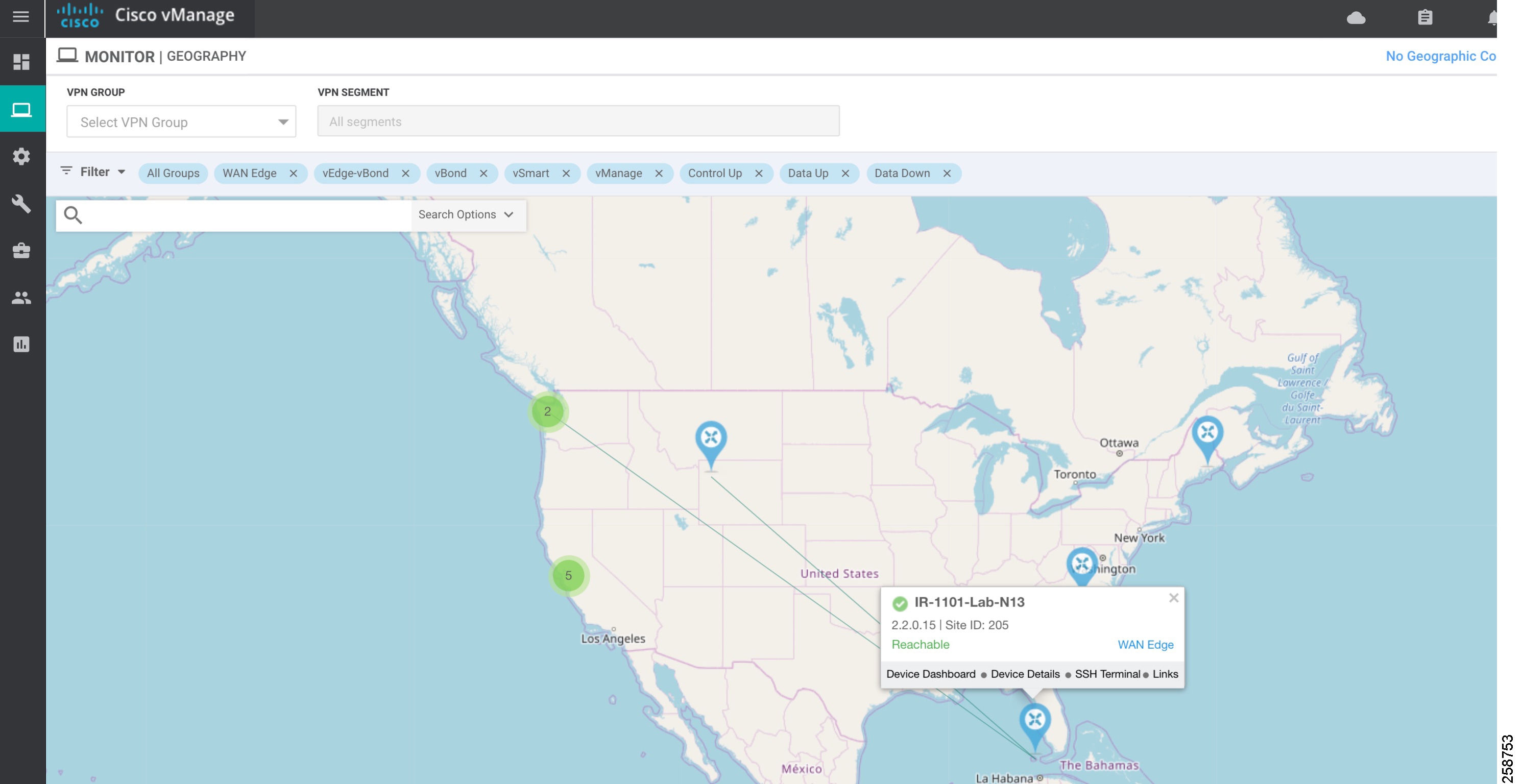This image depicts the Cisco vManage interface, a centralized network management tool used for configuring, monitoring, and maintaining network infrastructure. The layout showcases a detailed and navigable interface. 

On the left-side navigation bar, several icons are displayed, including a computer screen, gear, wrench, box, people, and charts, indicative of various network management categories and functionalities. 

The primary section of the image features a comprehensive map of the United States extending into parts of Canada. The map is marked with various connection points ranging from Washington state to Florida, highlighting a network of interconnected sites. These network points are joined by lines, likely representing VPN connections or a server network layout. Each marked location appears to be part of a larger network group, possibly indicating server clusters or VPN hubs.

A specific pop-up detail near Florida provides precise information about the routing number, suggesting active monitoring or configuration in that area. 

At the top of the interface, there's a search bar along with filtering options, enhancing ease of navigation and functionality for network administrators. The presence of the 'VPN Group' label further supports the context of VPN or server group management.

Overall, the image illustrates an active session within Cisco vManage, showcasing the geographical distribution and real-time management of a network infrastructure.